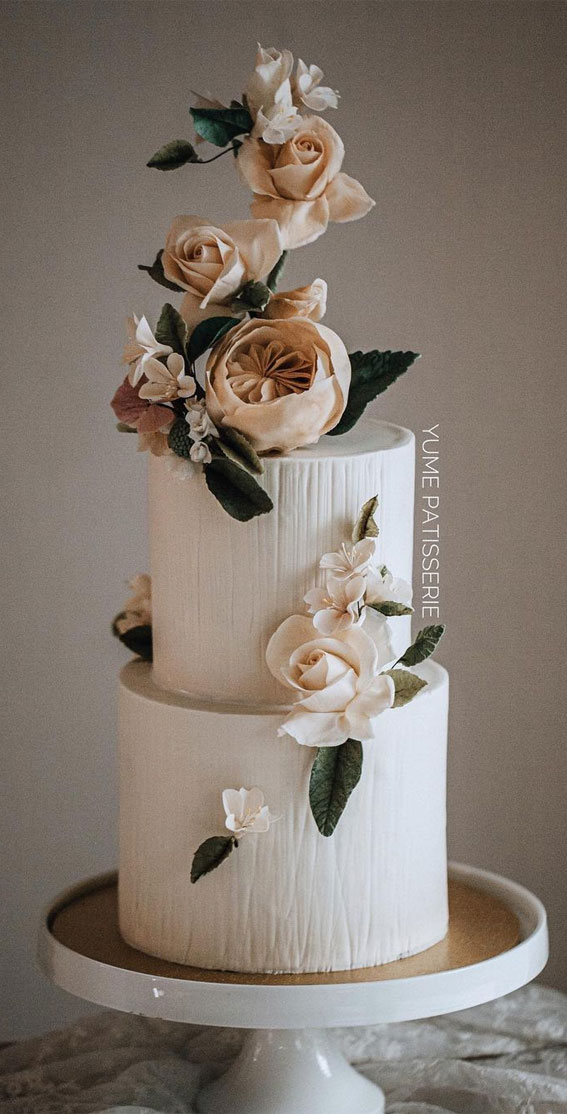This photograph features a stunning two-tiered wedding cake with intricate detailing. The layers of the cake are a pure white with textured vertical striations, resembling the bark of a tree, achieved through a fondant-style frosting. The cake rests on a sleek white pedestal cake plate, which has a golden brown base and a gold inlay, adding an elegant touch. 

The cake is adorned with delicate floral decorations: predominantly white roses, smaller white flowers, and green leaves that appear lifelike. These flowers cascade down the front and the left side of the cake. At the top, the floral arrangement transitions from the white flowers to include more pastel hues of beige and pink. A notable beige flower, possibly a peony, stands out among the green leaves and stems, creating a lush bouquet that extends above the top tier.

The background of the image features an ombre effect, transitioning from a medium-dark brown at the top to a light gray near the bottom, where it meets a white tablecloth or surface. Overlaying the image is a vertical logo that reads “Yume Patisserie,” indicating the bakery responsible for this beautiful creation. The overall composition of the photograph emphasizes the cake's elegant design and the artistry of its decoration.